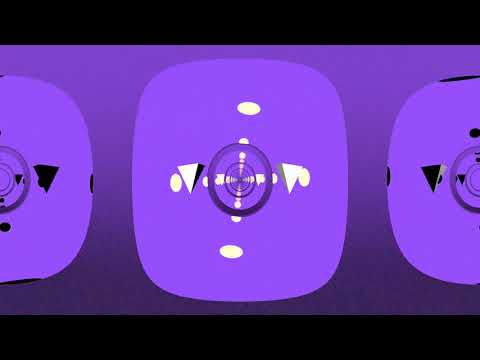This abstract art piece features a base background of a purple gradient, transitioning from a light purple at the top to a darker purple at the bottom. The image is encased with black borders on both the top and bottom. Centrally located in the composition, there are three uniquely shaped purple squares with rounded edges, resembling almost circular forms. The left and right squares are cut off halfway by the frame and are nearly identical in design. The center square is fully visible and distinctively different; it contains a series of concentric circles, each progressively smaller, and is adorned with white geometric shapes — specifically, an oval situated at the top and bottom, and upside-down triangles flanking the sides. The left and right squares also feature similar compositions of triangles and circles but in black and gray tones. The entire image exudes an enigmatic and layered feel, blending assorted shapes and shades primarily in the purple and white color spectrum, accented by the structured black borders.